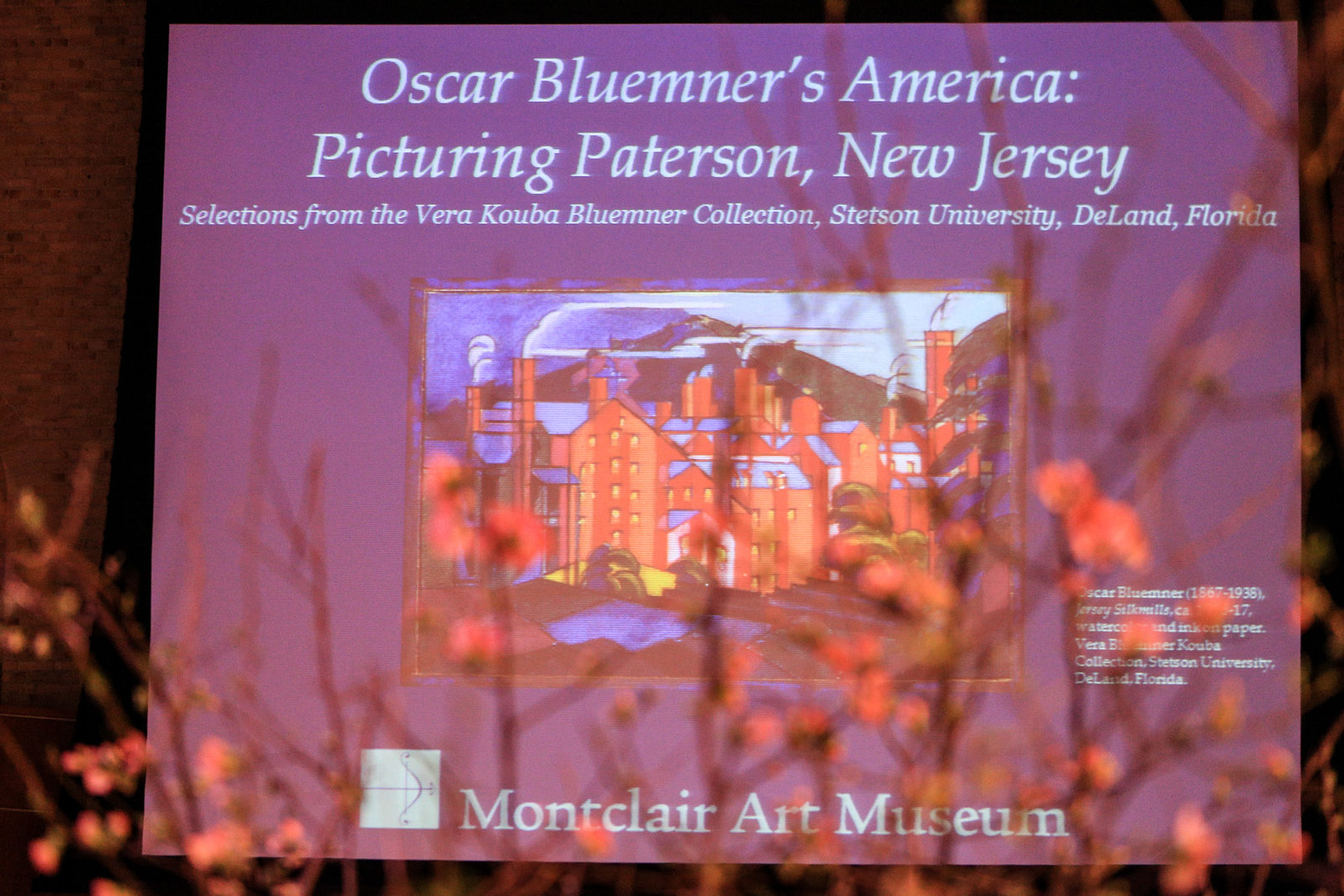The image depicts a poster advertisement with a predominantly purple background. At the top, white letters spell out "Oscar Blumner's America: Picturing Paterson, New Jersey". Below this, in smaller text, it reads, "Selections from the Vera Kuba Blumner Collection, Stetson University, DeLand, Florida." The central portion features a slightly abstract, possibly Cubist-style drawing of several orange buildings with numerous chimneys emitting smoke. The bottom of the poster states "Montclair Art Museum" in white letters. The scene is set in a dark environment, either outdoors or an event space, with brown branches bearing orange-pink buds partially obscuring the view, giving the image a sense of depth. The overall atmosphere combines the detailed artwork and text into an eye-catching display.